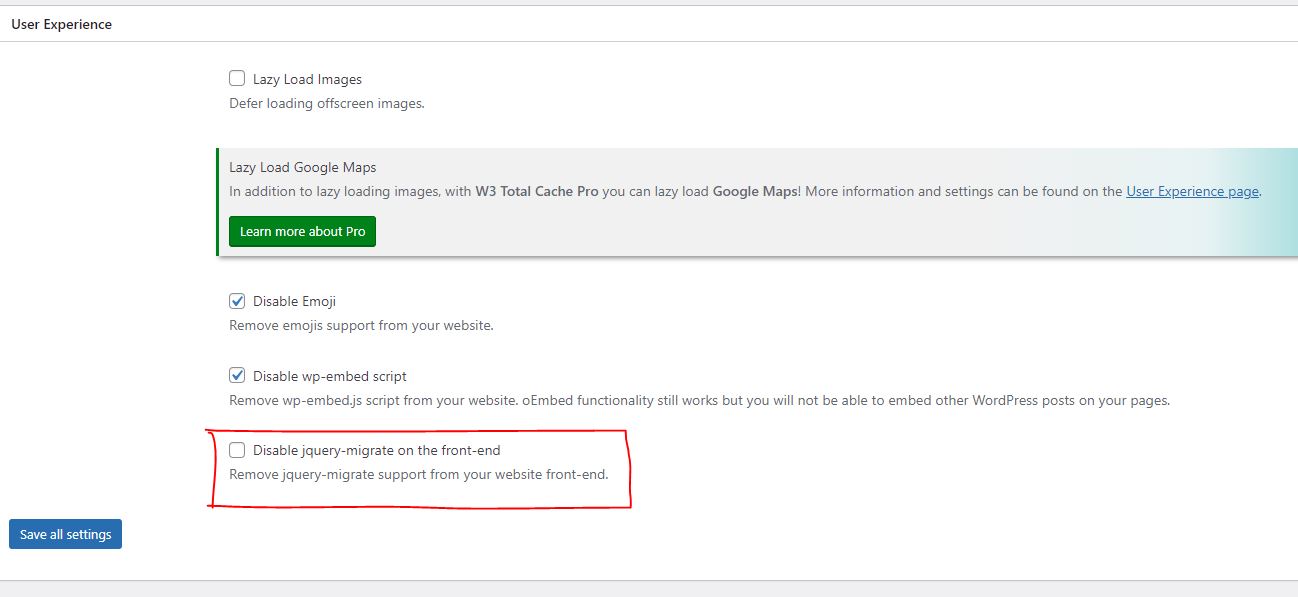The image displays a customization tab with several settings related to user experience. At the top left corner, there is a label that reads "User Experience." Below this, towards the middle, a white box is labeled "Lazy Load Images." Directly beneath this is another option, saying "Defer Loading Off-Screen Images." 

Next, there is a gray box that provides additional functionality, titled "Lazy Load Google Maps." The accompanying description states, "In addition to lazy loading images with W3 Total Cache Pro, you can lazy load Google Maps. More information and settings can be found on the User Experience page."

Towards the bottom of this section, a green button is displayed with the text "Learn More About Pro." Lastly, at the very bottom of the tab, there is a box with an option labeled "Disable Something Migrate Front-End."

The layout clearly categorizes different lazy loading and deferred loading options aimed at improving user experience, along with pointers to additional resources and settings.